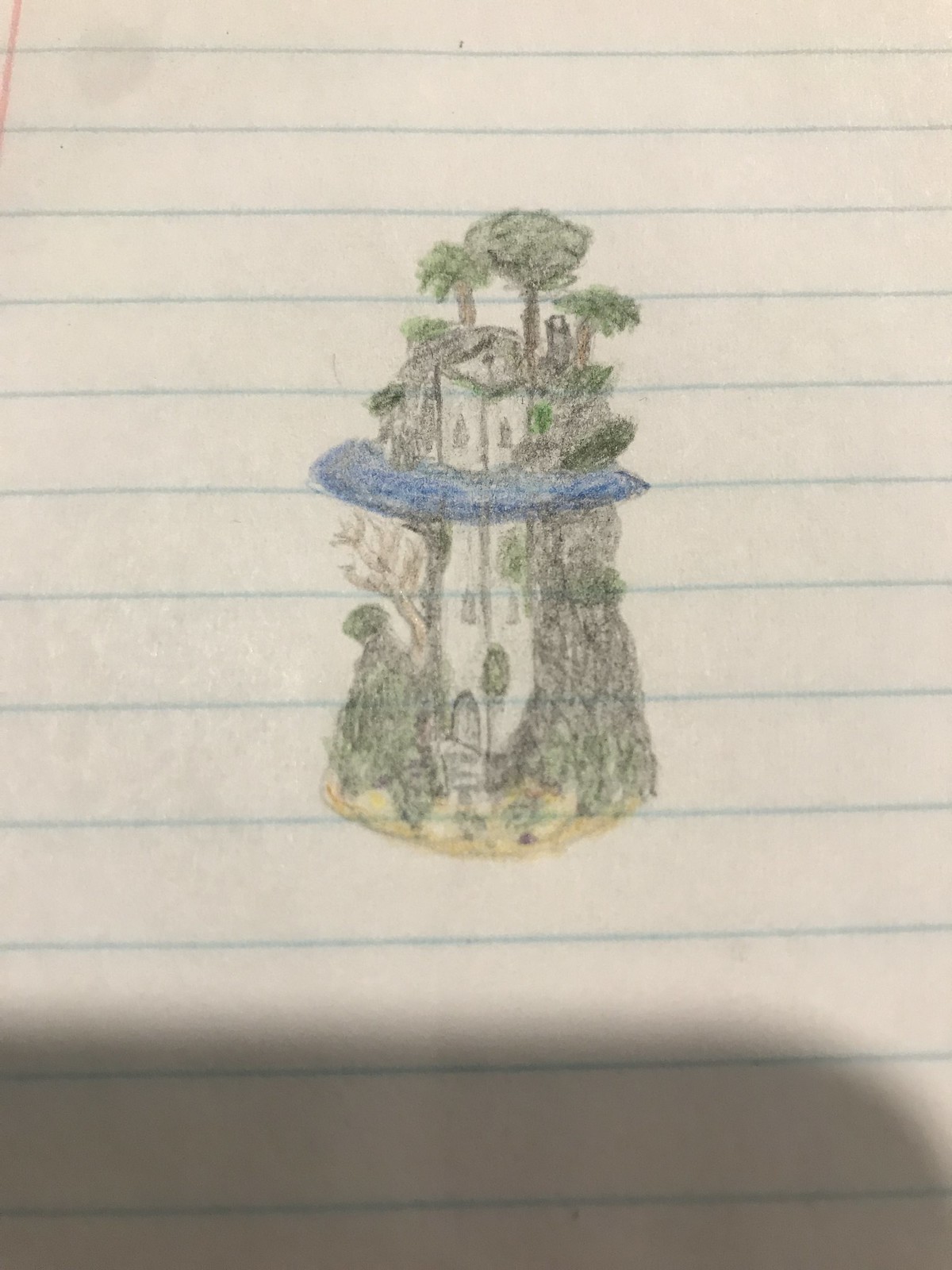This is a detailed pencil and colored pencil sketch on wide-lined, notebook paper characterized by its blue lines. The drawing itself is of a tall, slender tower-like house or castle built into a mountainous landscape. This building, depicted in black and white, has a series of windows and a prominent arched doorway at its base, suggesting a potential for an elevator or stairway inside. The structure appears cylindrical and lacks a roof, enhancing its tower-like appearance.

Surrounding the building is a mountain, shaded in dark pencil, which features a variety of greenery. Trees and shrubs populate the mountain, with some trees halfway up the left side and several situated at the peak, displaying green foliage and brown trunks. A striking blue border or platform encircles the top of the mountain, resembling water, adding an element of surrealism to the image.

Across the entire bottom quarter of the page is a shadow, presumably cast by someone holding the paper. This shadow angles downwards from the left until it exits the page on the right. The combination of meticulous pencil shading and light green accents in the foliage provides the sketch with a depth and texture that brings the imaginary scene to life.